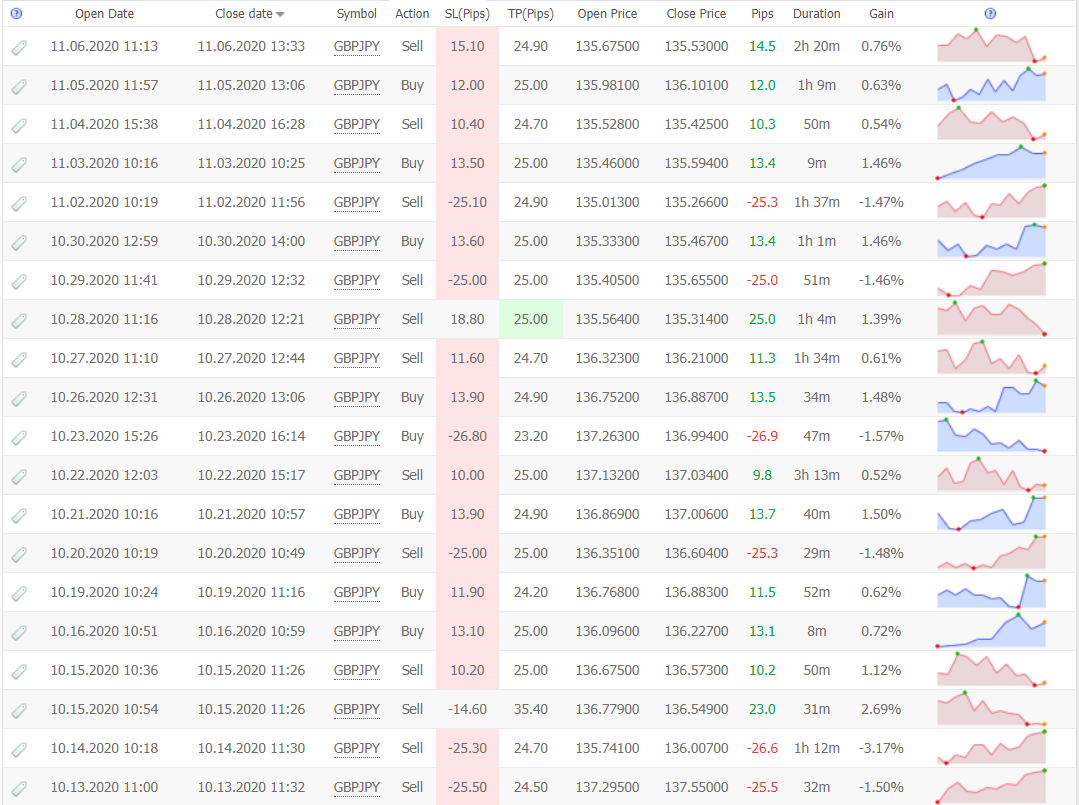This detailed screenshot captures the active trading positions of an individual engaged in Forex trading, specifically focusing on the British Pound (GBP) versus the Japanese Yen (JPY). The data is presented in a comprehensive table format, featuring over 20 rows and more than 10 columns, meticulously charting the trades. The columns, clearly labeled, include: Open Date, Closed Date, Symbol, Action, SL Pips, TP Pips, Open Price, Closed Price, Pips, Duration, and Gain. Additionally, there is a graphical element depicting the price action.

Examining the open and closed dates, it is evident that the trades predominantly took place in October and November of 2020. The consistent symbol across all rows is GBP/JPY, indicating a focused trading strategy on this currency pair. The trader has engaged in a mix of buying and selling actions, with performance metrics showing a tendency towards modest gains, predominantly in the range of 0.3% to 1.5%. The first four trades depicted show gains, followed by a loss on the fifth trade, and this gain-loss pattern appears to persist throughout the dataset. The background of the table and charts is white, providing a clean and clear view of the trading data.